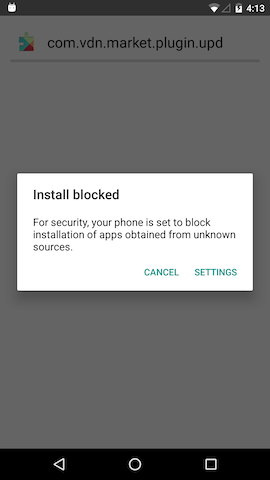The image is a screenshot of a smartphone screen with an overall dark gray overlay, giving it a grayed-out appearance. The original background seems to be white but is dimmed by the overlay, making the elements on the screen more pronounced.

At the very top of the screen, there is a black banner. On the left side of this banner, there is a small, somewhat indistinct icon that may resemble a calendar. The right side of the banner displays typical smartphone status icons: wireless availability, signal strength, and a vertically-oriented battery icon indicating approximately 90% charge. Adjacent to these icons is the current time, displayed in white font as "4:13".

Beneath this top banner, a colorful jigsaw piece icon in green, yellow, red, and orange is visible next to a string of text that reads, "COM.VDN.VDN.Market.Plugin.UPD."

Dominating the center of the screenshot is a prominent white rectangular notification box with black trim. The content within this box is critical information regarding app installation. Bold black text at the top of the box reads "Install Blocked." Below this, in smaller gray text, is a message explaining the block: "For security, your phone is set to block installation of apps obtained from unknown sources."

At the lower right corner of the notification box, two green capitalized options are available: "CANCEL" and "SETTINGS."

Finally, at the very bottom of the screen, another black banner contains the smartphone's navigation icons. From left to right, these icons include a white triangle pointing left (back), a white circle (home), and a white square (recent apps).